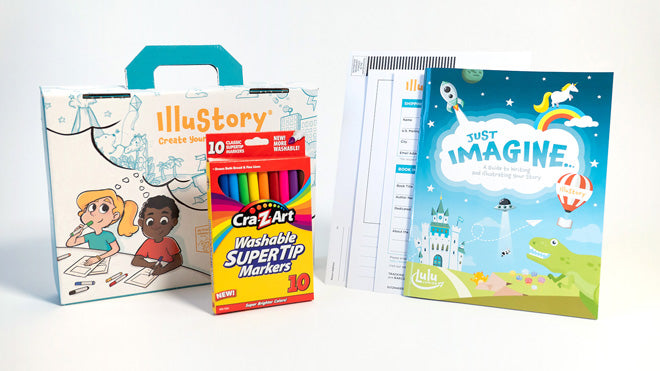The photograph showcases a selection of children's stationary items arranged on a white tabletop with a white wall background. To the right side of the image, there is a blue and green book titled "Just Imagine," adorned with vibrant illustrations of a castle, a reptile, a hot air balloon, a rainbow unicorn, a spaceship, planets, stars, kites, and bees. Centrally positioned is a white rectangular object, possibly a form or booklet. To the left is a white briefcase-like painting book with a blue handle, labeled "Illustory," featuring animated drawings of a boy and girl engaged in creative activities with crayons. The briefcase cover has a playful design with animals and buildings. In front of the briefcase is a yellow and orange box of Cra-Z-Art Washable SuperTip Markers, boasting the tagline "10 Classic SuperTip Markers – New, More Washable." The markers inside are displayed in an array of bright colors including blue, green, yellow, orange, red, pink, purple, and violet, visible through the transparent front. The scene is a delightful display of art supplies aimed at young children, ideal for fostering creativity and imagination.